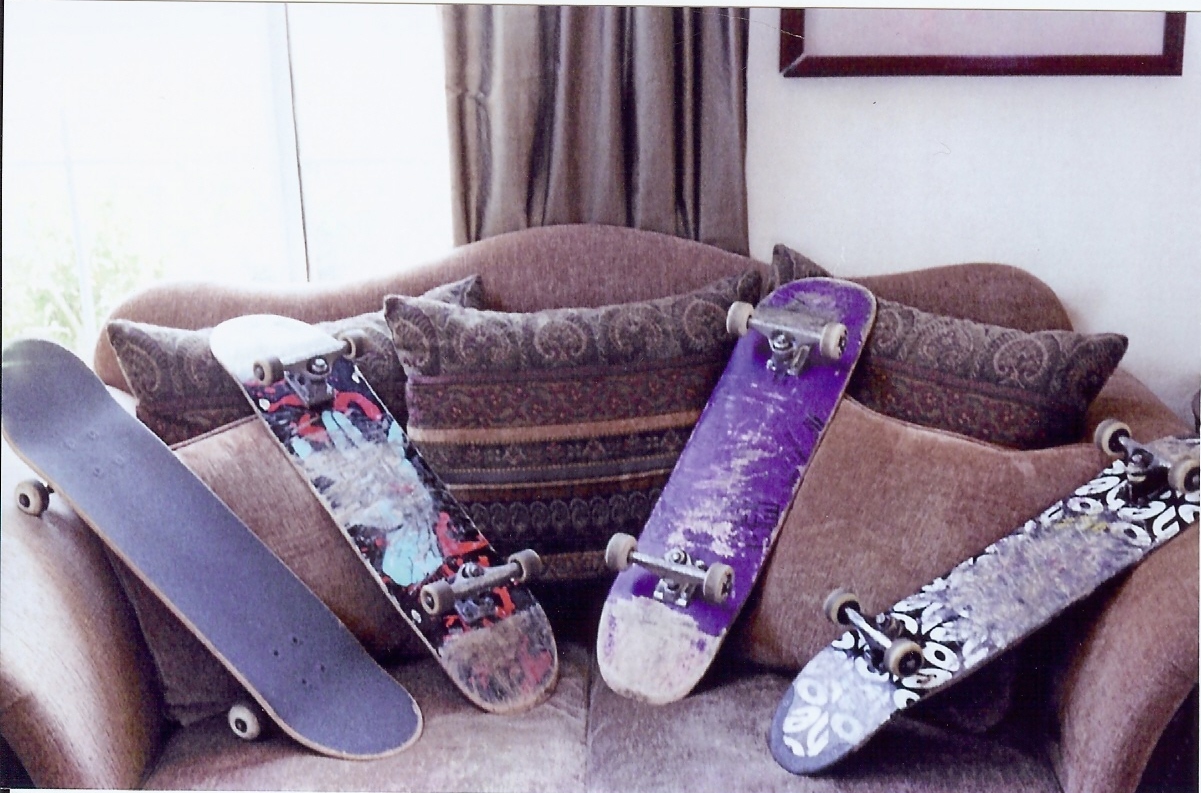The photograph captures a cozy indoor scene, featuring a brown couch adorned with five large pillows, three of which have decorative designs of lines and shells. The couch is situated against a white wall, with brown curtains partially drawn open, allowing bright sunlight to filter in and highlighting a glimpse of greenery outside the window. A picture with a brown frame hangs on the wall beside the window. 

On the couch, four well-used skateboards are meticulously arranged. The skateboard on the far left is black and faces upwards, displaying its plain deck. The second skateboard rests on its back with its wheels up, featuring a colorful, scratched-up design with red, blue, and black elements. The third skateboard, also lying wheels-up, has a purple and white deck, similarly showing signs of wear. The fourth skateboard, positioned on its back with its wheels up as well, showcases a black deck with white letters all over it. The skateboards' dirty white wheels and silver hardware indicate heavy usage, adding character to the overall scene. The photograph's background ambiance is further enriched by the large window allowing in ample daylight, accentuating the earthy tones and relaxed atmosphere of the room.